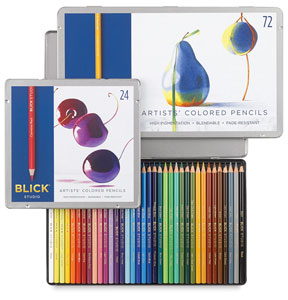This image showcases a vibrant array of colored pencil boxes arranged on a white background, featuring an artistic and detailed depiction of their contents. Dominating the front left section is a square box labeled "24" from the brand Blick. The box features an illustration of cherries in various hues, ranging from dark purple to a more traditional cherry red. This box also has a blue section with a red colored pencil displayed prominently. Just behind this is a larger box stating "72" in blue text, marked as "artist colored pencils" with a striking illustration of a multicolored pear, blending shades of blue, green, yellow, and orange, and accented by a green leaf.

Below these main boxes is an open lid showcasing a collection of colored pencils from the "72" kit, arranged to display a spectrum that includes every color in the rainbow: whites, yellows, oranges, reds, purples, pinks, teals, blues, light and dark greens, and various browns. In the backdrop of this collage is a small gray rectangular element, subtly enhancing the composition's depth and balance.